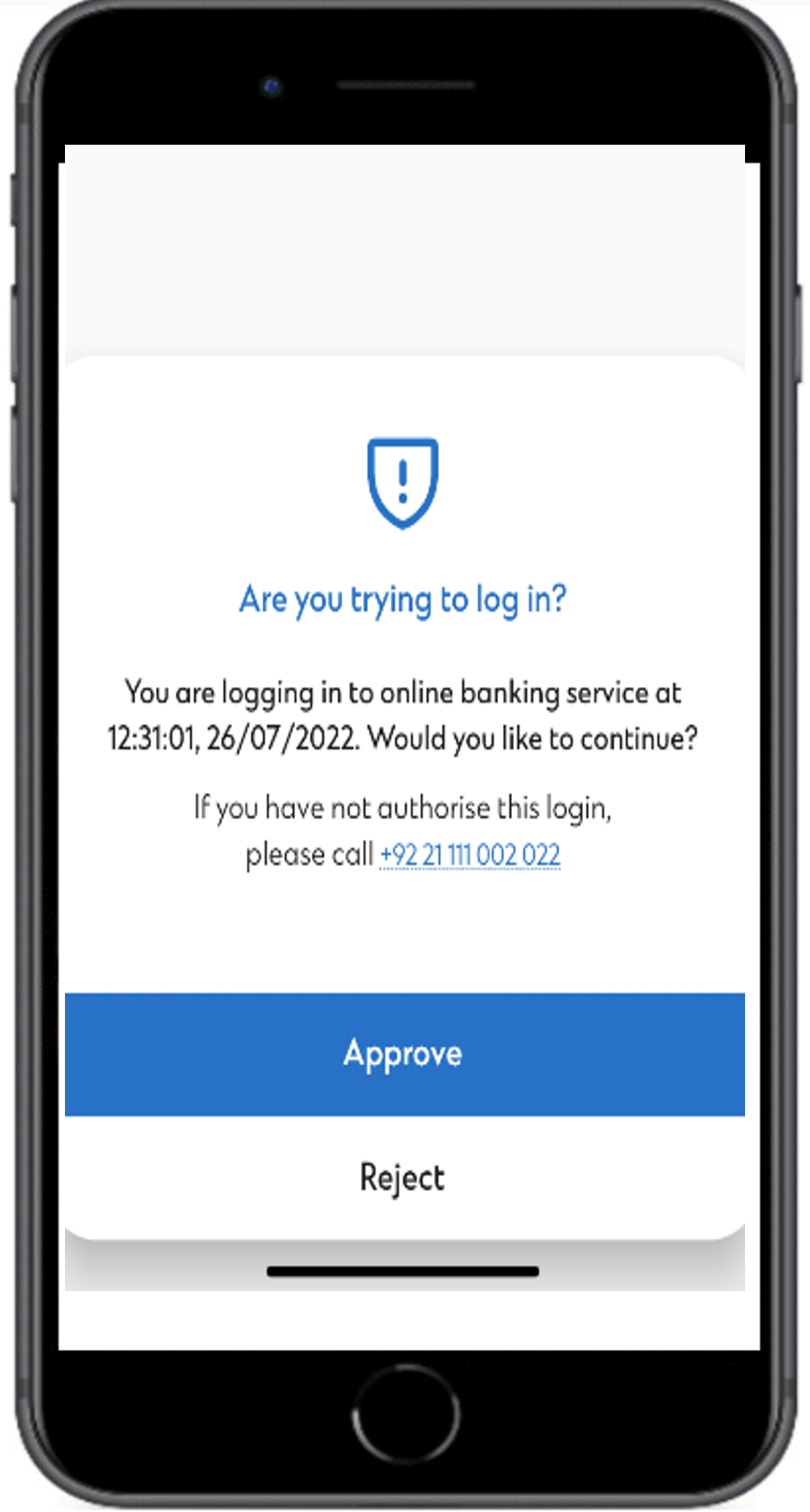The image depicts a black cell phone encased in a black physical case. The phone features slightly chrome-trimmed edges. On the left side of the device, there is a volume button, while the right side hosts what appears to be an on-off or home button. 

The phone's screen displays a predominantly white page bearing a distinctive upside-down shield logo in blue, with an eye in the middle. The center of the eye contains a blue exclamation point. Beneath the logo, the text reads, "Are you trying to log in?" followed by, "You are logging in to Online Banking Service at 12:31:01 on 26-07-2022." 

Further down, the text prompts, "Would you like to continue?" Below this message, there is a notice stating, "If you have not authorized this login, please call," followed by a contact number. At the bottom of the screen, two buttons are visible: an "Approve" button and a "Reject" button.